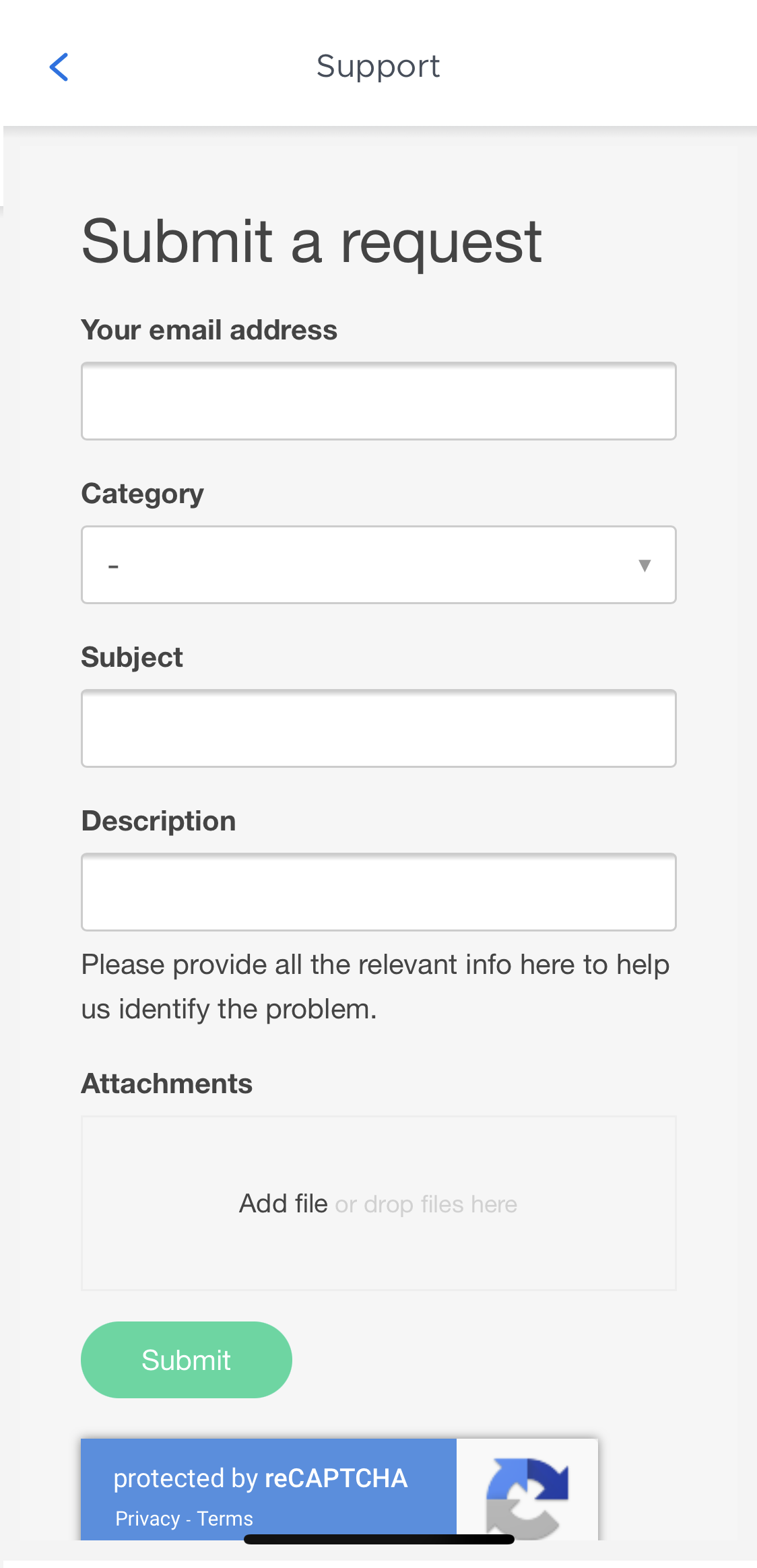This is an image of a mobile-friendly support request form designed for both smartphones and tablets. At the top of the form, there is a distinctive "V" shaped arrow icon pointing to the left, followed by the word "Support" in light gray text. Below this header, the background shifts to a light gray color with black text, featuring the header "Submit a Request."

The form itself consists of four input fields: 
1. Email Address
2. Category
3. Subject
4. Description 

A message underneath these fields urges users to "Please provide all the relevant info here to help us identify the problem." Below, there is an "Attachments" section where users can upload files. This section includes a smaller rectangle with the text "Add File" in black, accompanied by a lighter gray message that reads "or drop files here."

At the bottom left corner of the page, there is a green button labeled "Submit" in white text. The page’s footer indicates that it is protected by reCAPTCHA, with links to "Privacy" and "Terms" policies.